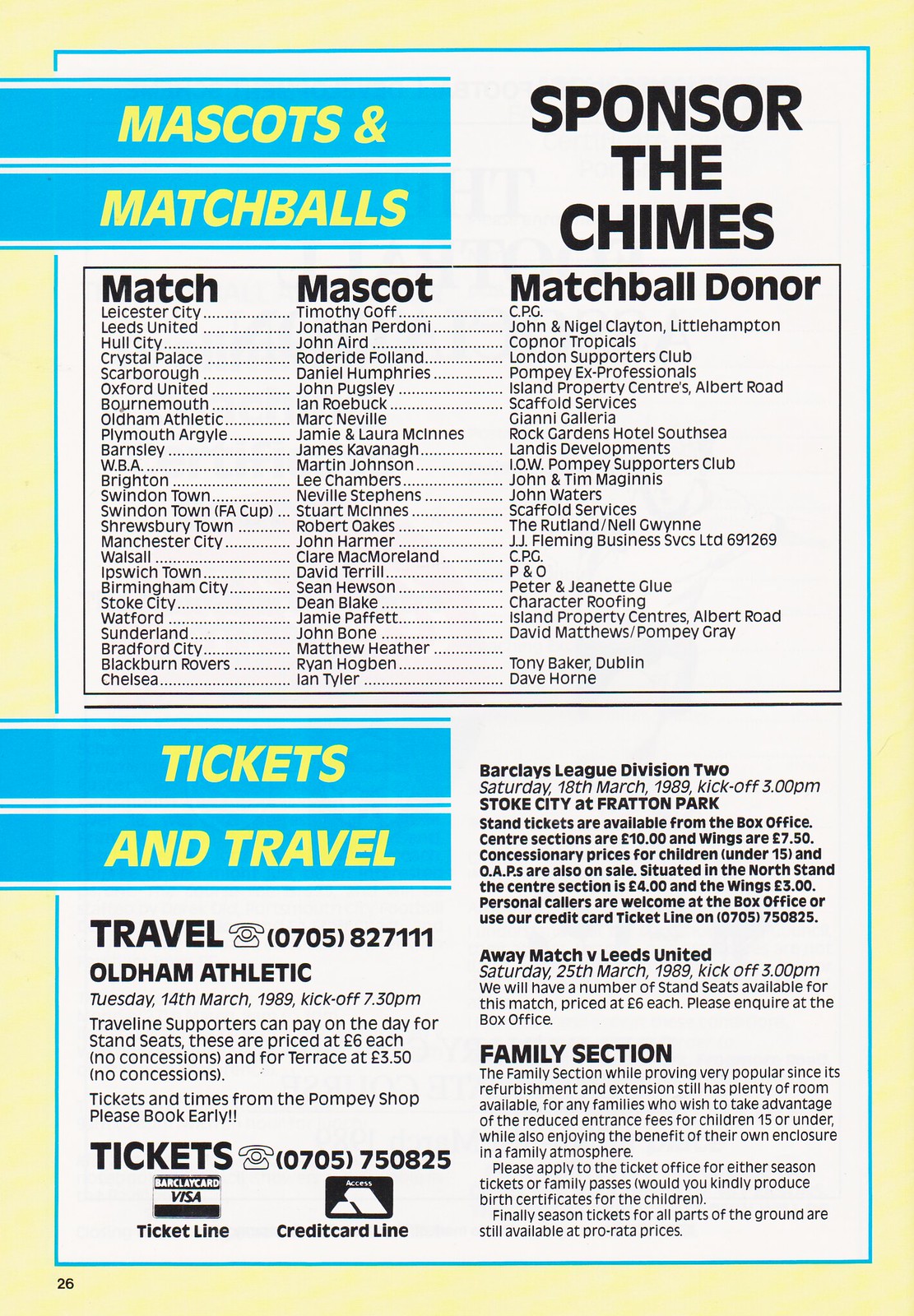The image resembles an advertisement or flyer with a yellow border, a thin blue border inside it, and a white background. At the top left, it features a blue bar with yellow text that reads "Mascots and Match Balls." Adjacent to this, on the top right, it says "Sponsor the Chimes" in black letters. Below these headings is a detailed chart with three columns labeled "Match," "Mascot," and "Match Ball Donor," listing specific names and sponsors. Further down, another blue bar with yellow text reads "Tickets and Travel." The section beneath provides extensive travel and ticket information in black text, including pricing, dates, and family section details. This section includes a phone number (0705-827-111), dates such as Tuesday, 14th March 1989 with a kickoff at 7.30 PM, and mentions the availability of season tickets. Payment methods like Visa and Credit Card are indicated with logos. The entire layout is meticulously designed to offer clear and comprehensive information about match sponsorship, tickets, and travel arrangements.